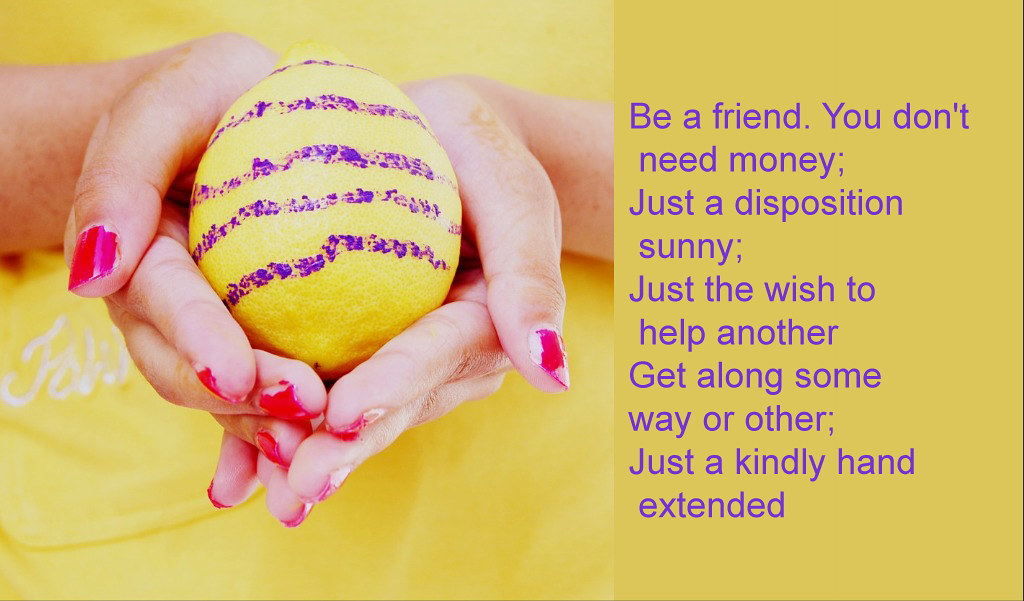In this promotional full-color image, which appears to resemble the front of a postcard or greeting card, the central focus is on a Caucasian woman's hands. Her hands, adorned with chipped red nail polish, are prominently displayed holding a bright yellow lemon that features purple stripes drawn around it. The background is a dominant, dark mustard yellow without any visible border. To the right of the delicately cradled lemon, there is a motivational inscription rendered in purple print. It reads: "Be a friend. You don't need money, just a disposition sunny. Just the wish to help another get along some way or other. Just kindly extend a hand." Additionally, some white lettering, seemingly consisting of an 'F', an 'A', and a 'K', is faintly visible at the far lower left corner. The entire composition exudes a cheerful, inviting atmosphere with its vivid colors and uplifting message.